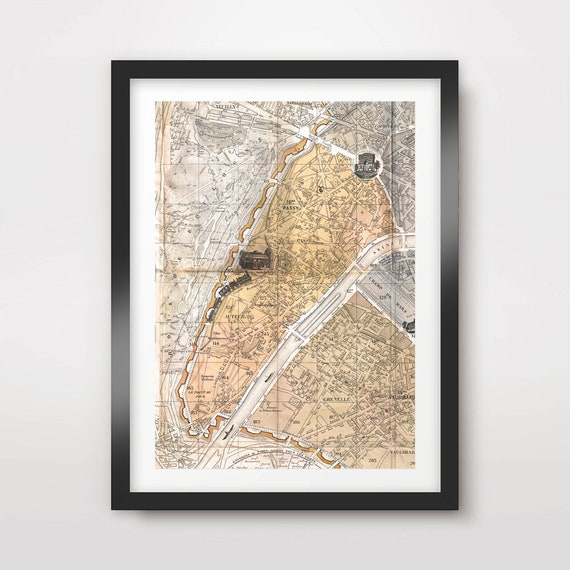The photograph depicts an old-fashioned map framed in a plain brown frame with a white mat, set against an off-white wall. The map features intricate details, making it difficult to pinpoint the exact location, but it shows a top-down view of a city's layout with roads, highways, and side streets distinctly marked. The map employs a palette of beige, tan, cream, and black, with different shadings segregating various territories. Prominently, there is a large black structure in the center, possibly an important building, and a circle containing text that might denote a significant landmark. Among the text visible on the map is the word "SEINE," suggesting that this map represents a region in France. The map also includes thin grid lines forming squares across its expanse and an illustration of several train cars, indicating a railroad. Although the map's origin is uncertain—whether it’s a hand-drawn sketch or a computer-generated print—it captivates with its detailed and historical appearance.